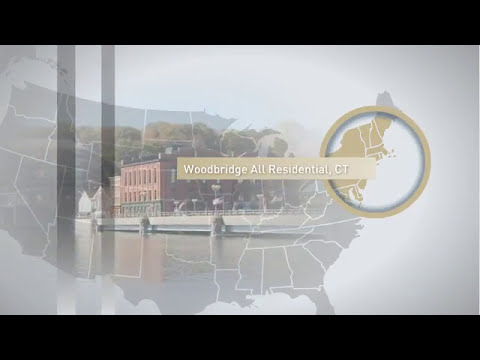This image features a gray map of the United States, with white lines delineating state borders. A magnified section in the top-right corner highlights the northeastern states, prominently displaying them in a tannish hue. A rectangular box with white text reads "Woodbridge All-Residential Connecticut." Overlaid on the map is an image showing a serene body of water beside a large brick building, which appears to be a central structure in the residential area of Woodbridge, Connecticut. The setting includes a deck with an outdoor eating area, possibly captured from a boat. Additional small buildings with A-frame roofs, one white and one red, are visible in the background amidst lush green trees. Black borders frame the top and bottom of the image, suggesting it may be part of a presentation slide showcasing this picturesque location. The colors in the image include black, gray, brown, tan, green, white, yellow, and gold, bringing the tranquil Connecticut setting to life.